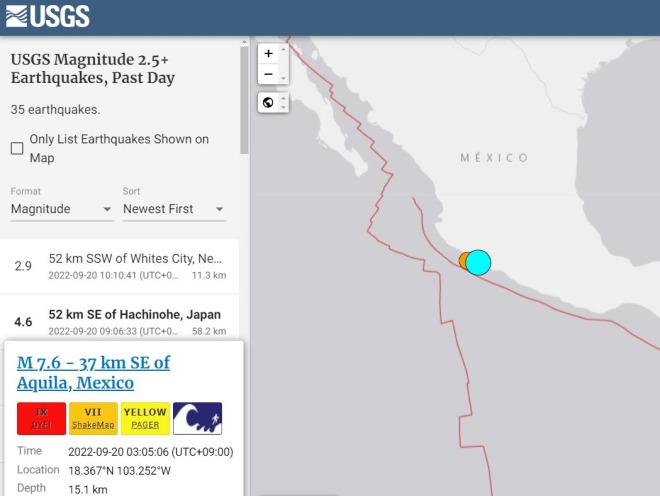This is a screenshot from the USGS website, featuring a dark bluish-gray banner at the top that prominently displays "USGS" in white letters. Below the banner, on the left side, there's a section titled "USGS Magnitude 2.5+ Earthquakes, Past Day," indicating there are 35 earthquakes recorded in the past day, though the checkbox for "Only List Earthquakes Shown on Map" is not checked. The earthquakes are sorted by magnitude and displayed in descending order. 

Details include:
- A magnitude 2.9 earthquake located 52 km SSW of White City, NE, occurring on September 20, 2022, at 10:10:41 UTC at a depth of 11.3 km.
- A magnitude 4.6 earthquake located 52 km SE of Hachinohe, Japan, occurring on September 20, 2022, at 09:06:33 UTC at a depth of 58.2 km.
- A significant magnitude 7.6 earthquake situated 37 km SE of Akiwa, Mexico, recorded on September 20, 2022, at 03:05:06 UTC, with a time difference of +09:00 UTC, positioned at 18.367 degrees north and 103.252 degrees west, with a depth of 15.1 km.

On the right side of the screenshot, there is a gray and white map depicting Mexico. Notably, a turquoise-colored circle near the bottom edge of Mexico marks the location of the notable earthquake.